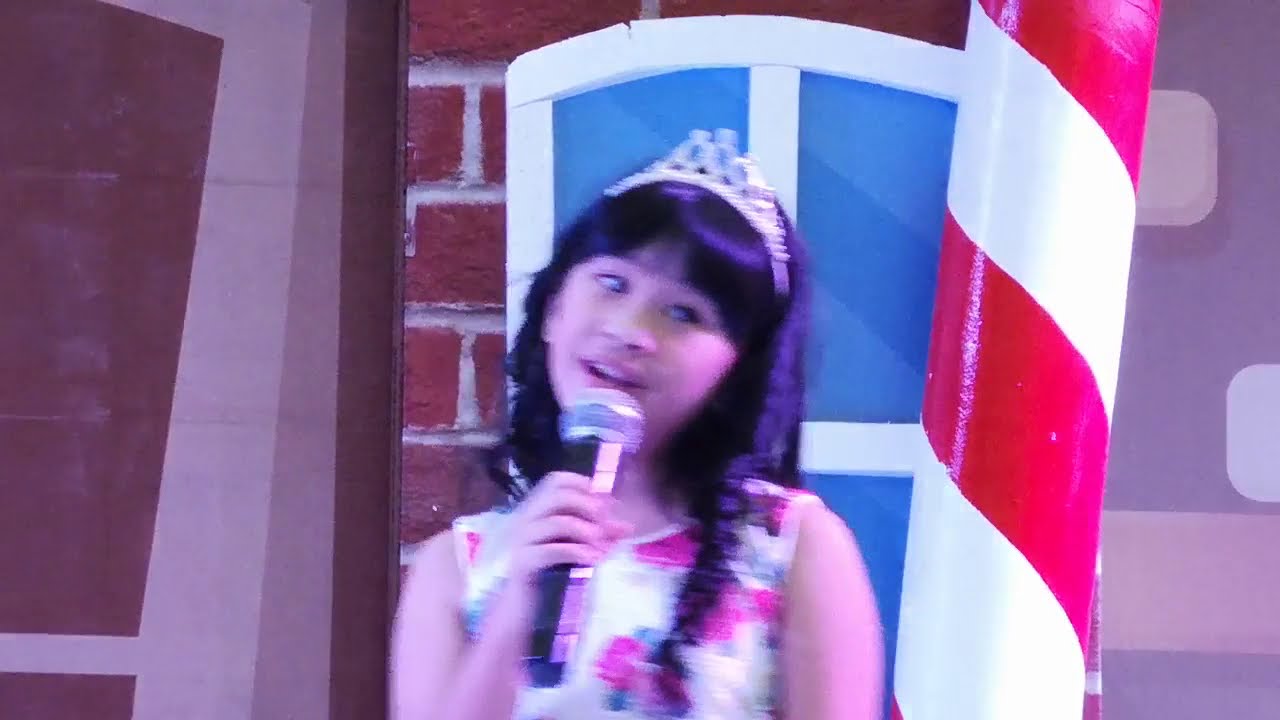In this somewhat blurry photograph, a young girl, around 10 years old, stands center stage, singing into a microphone with her mouth open. She has long, dark hair with bangs and wears a silver tiara on her head. Her attire is a sleeveless dress adorned with red flowers on a mostly white background. The image captures her from the chest up. To her right, a pole painted like a candy cane adds a festive touch, while directly behind her, a white-trimmed blue window and a backdrop of a painted brick wall create depth in the scene. The setting appears to be indoors, likely on a stage filled with props. The girl looks directly at the camera, embodying the focus of this charming theatrical moment.